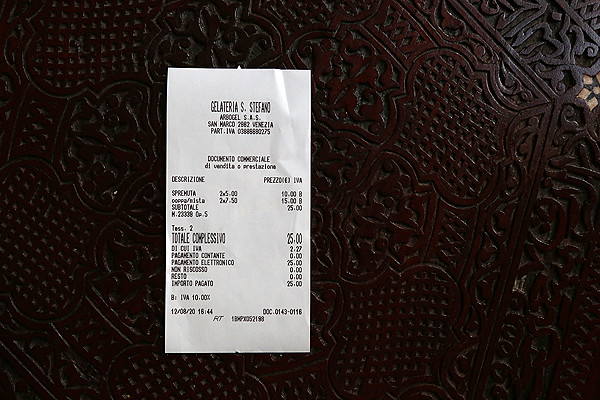This photo captures a somewhat out-of-focus receipt, printed on a small piece of vertically oriented white paper with black text that's difficult to decipher. The blurred text suggests it might be from an Italian establishment, potentially referencing a name like "ga-gel-otarius" or something similar, though it's not entirely clear. The receipt sits upon a beautifully ornate, brown carved surface that appears to be part of a table. This backdrop features an intricate design reminiscent of Moroccan lamp shapes, adorned with small diamond indentations. The rich, chocolate brown color of the table adds a touch of elegance to the scene.